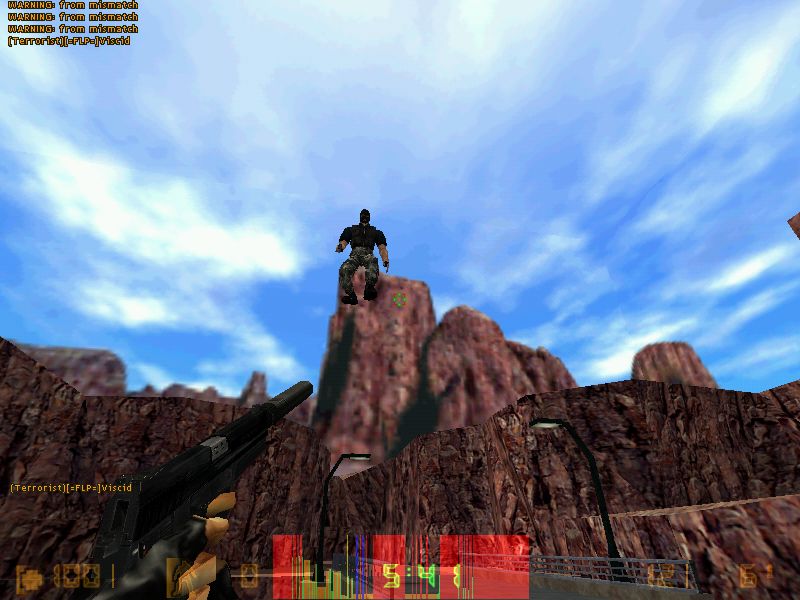The image is a detailed screenshot from a first-person shooter computer game, set in a rugged, rocky landscape reminiscent of a state park in Utah with striking red mountains. In the lower part of the image, jagged rock formations dominate the scene, while the upper two-thirds features a vivid sky, transitioning from light to dark blue, dotted with moving white clouds.

Positioned at the center of the image is a muscular character in camouflage pants, black boots, a short-sleeved black shirt, and possibly a black mask or helmet. This character appears to be floating in mid-air, in front of a rocky outcrop, adding a surreal element to the scene.

At the bottom of the screen, a digital timestamp reading "5:41" in yellow and green lettering indicates in-game time, possibly accompanied by a status bar displaying health or ammunition levels, although these details are hard to discern.

In the lower left corner, the gloved left hand of the player character extends into the frame, aiming a large black machine gun at the floating figure, suggesting imminent action. The tension is heightened by text overlays: "Warning from Mismatch, Warning from Mismatch" repeated in the upper left corner, likely indicating an in-game alert or potential communication between players. Additional text, "Terrorist FLP this sid," appears both here and closer to the bottom of the image, hinting at the storyline or mission objectives within this online multiplayer environment.